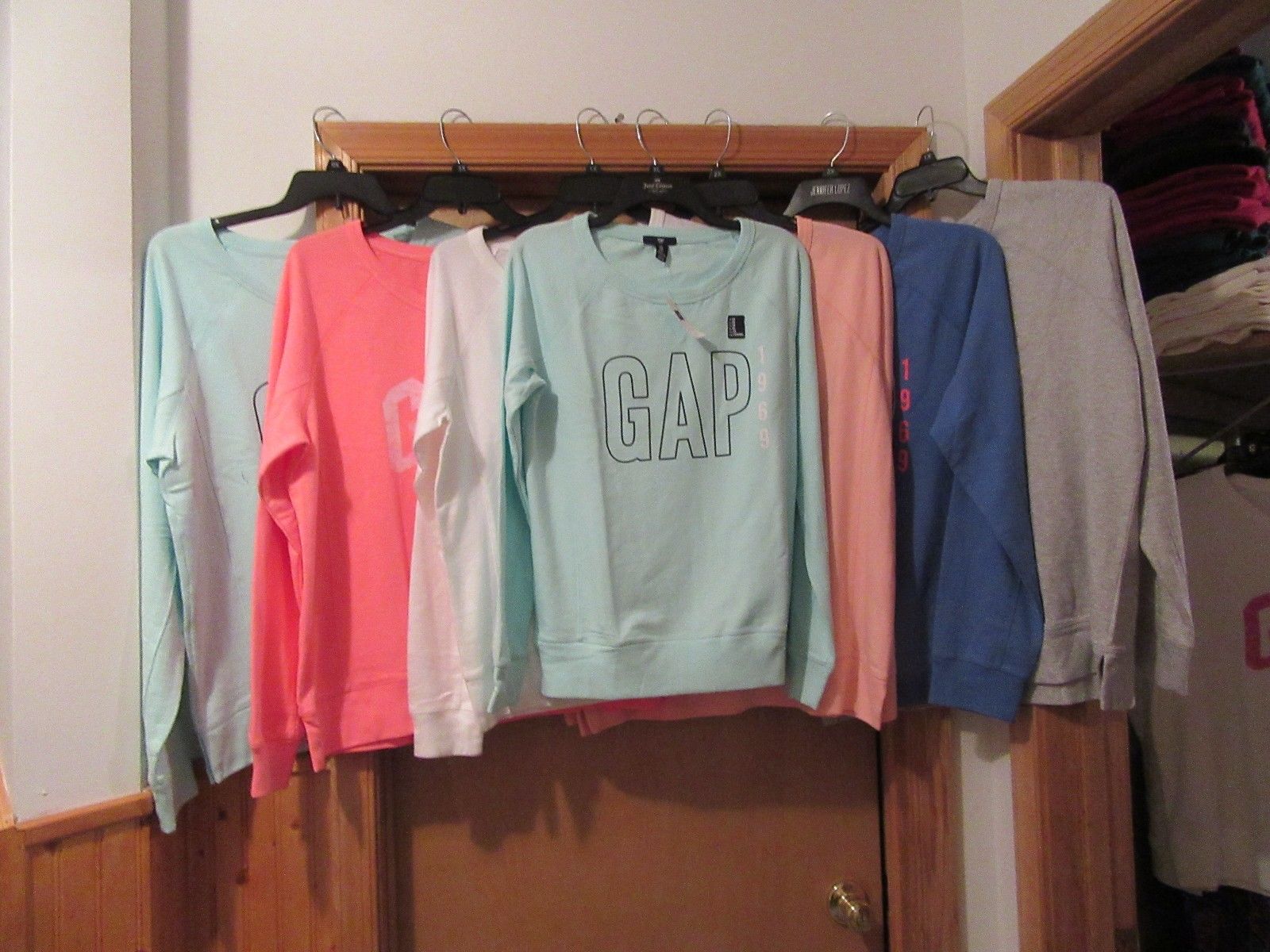This photograph depicts a wooden door with a gold doorknob, almost completely shut, with seven long-sleeve shirts hanging from black hangers on the top part of the doorframe. The wall to the right of the door consists of brown wooden paneling on the lower half and white plaster above. Adjacent to the door is an open closet revealing more hanging clothes and items stacked on a top shelf. 

The shirts on the doorframe are of various colors and the same design, each with the word "GAP" on the front. Starting from the left, we see a whitish pink shirt, a bright pink shirt, and a light blue shirt. In the center is a turquoise blue shirt with the word "GAP." To its immediate right, there is another pink shirt, followed by a royal blue shirt with additional designs in orange, and finally a gray shirt. These shirts appear to be uniformly sized and add a vibrant array of colors against the subdued tones of the wooden door and paneling.